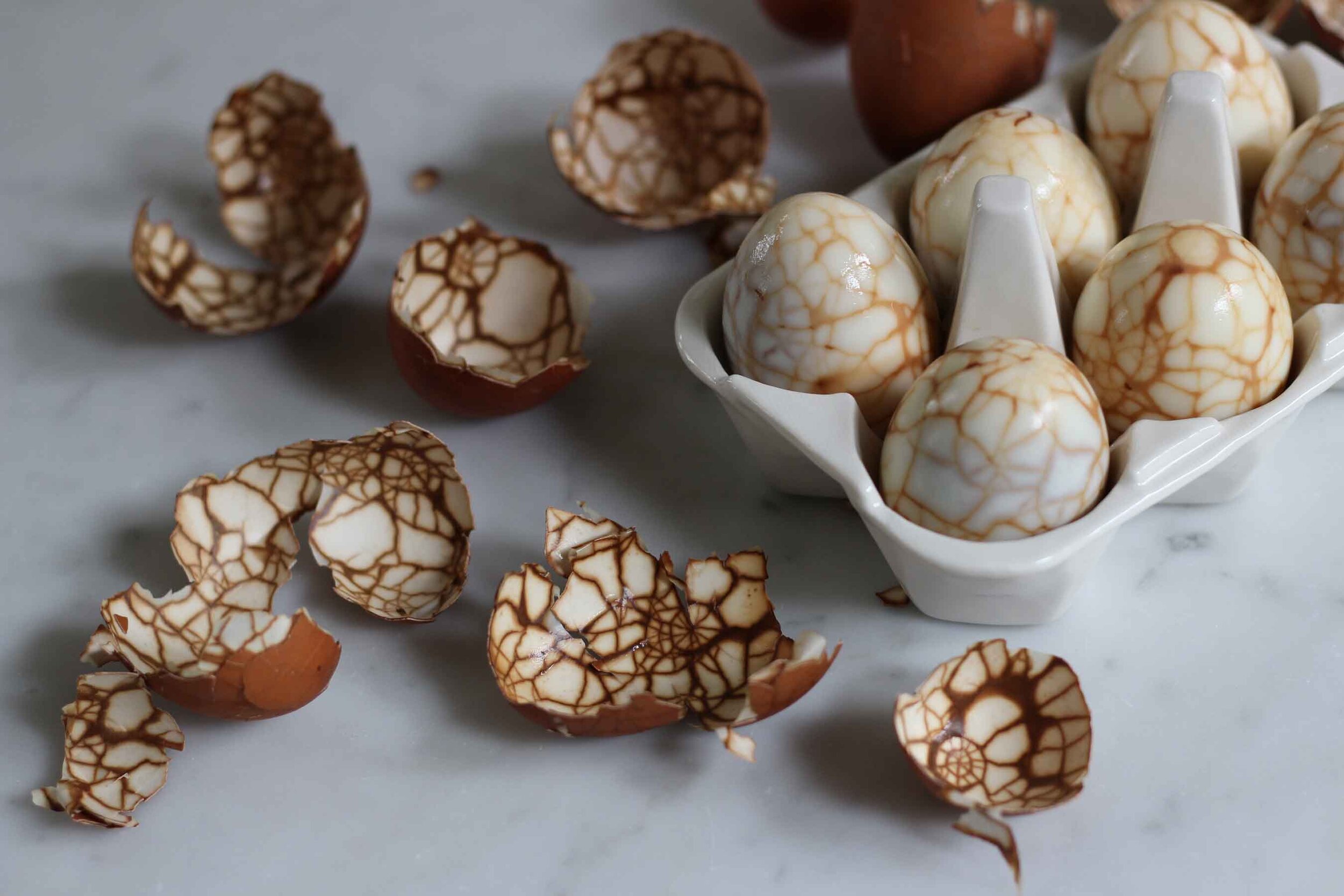The image depicts a carton containing six peculiar white eggs that appear to have a cracked, brown-veined pattern across their surfaces, giving them a distinctive, almost dinosaur-like appearance. The carton, set upon a white surface, is surrounded by several broken eggshells exhibiting the same crackled brown pattern on both their interior and exterior. It appears the eggs have been boiled and then peeled, with the unique veining possibly resulting from a boiling process where the shells were cracked and maybe treated with a substance like iodine, leading to the unusual texture and coloration visible on the eggs.